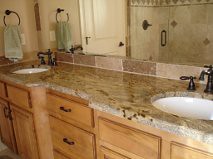This indoor close-up photograph features a beautifully designed bathroom vanity with two distinct sink areas. One sink is positioned in the far background on the left, while the other is prominently displayed on the right in the foreground. The photograph is captured at a slight angle, offering a comprehensive view of the vanity.

The cabinetry beneath the countertop boasts a light wood finish, enhanced by a central column of drawers that feature sleek black horizontal handles. The countertop itself is made of grayish-green marble interspersed with specks of brown, adding a touch of elegance to the space. Both sinks are equipped with black faucets that include separate simple horizontal levers for hot and cold water.

In the upper left corner of the image, a wall-mounted rack or loop holds a green hand towel, adding a pop of color. The towel extends from the background and trails out of frame toward the foreground. On the right side of the image, a large mirror spans the area, reflecting elements such as the bathroom door, centrally located in the reflection, and the bathtub with its light green tile, positioned slightly right of center.

The countertop is notably clear of any items, ensuring an uncluttered and streamlined look. The entire scene is well-lit and captured in decent focus, emphasizing the clean and sophisticated design of this bathroom vanity. No text, words, or print are visible within the photograph, maintaining the visual focus on the design elements.